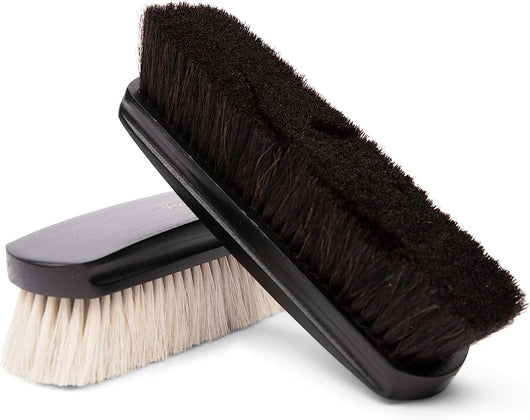This image features two long brushes against a white background. Both brushes have sleek, shiny black handles, and appear to be made of black wood. The brush on the left has thick brown bristles, while the one on the right has thick white bristles. The brown-bristled brush is leaning against the white-bristled one, creating a subtle interplay of colors and textures. The specific use of the brushes is unclear, but they may be designed for light brushing tasks, possibly for grooming animals or for cleaning items like shoes. The bristles on both brushes are relatively soft, adding to the ambiguity of their exact purpose.